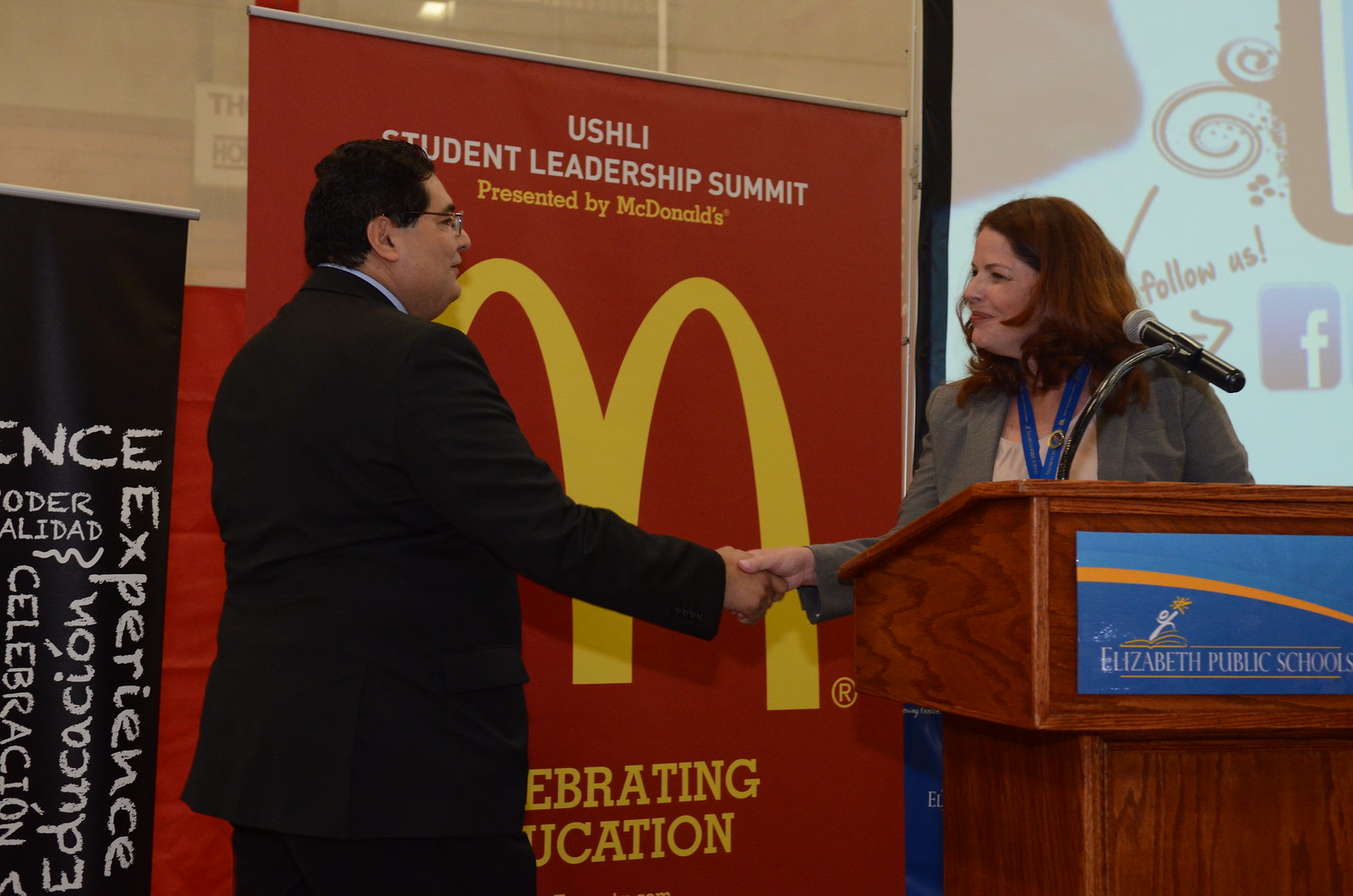In this image, two people are on a stage engaging in a handshake. The person on the left is a man with short black hair, wearing glasses and a black suit. His right arm extends to shake hands with the woman on the right, who stands behind a wood podium adorned with a blue plaque reading "Elizabeth Public Schools." The woman, with shoulder-length brown hair, wears a gray jacket over a light-colored cream top, and a blue lanyard around her neck. A microphone extends from the top of the podium towards her. Behind them is a large red banner with a prominent yellow McDonald's logo and white text that reads "USHLI Student Leadership Summit, presented by McDonald's, celebrating education." Additionally, a black banner with white writing is visible on the left side of the image. In the background, there is a screen with a Facebook logo and the text "Follow Us," along with another partially visible banner featuring the word "Experience." The setting appears to be an award ceremony or public speaking event.